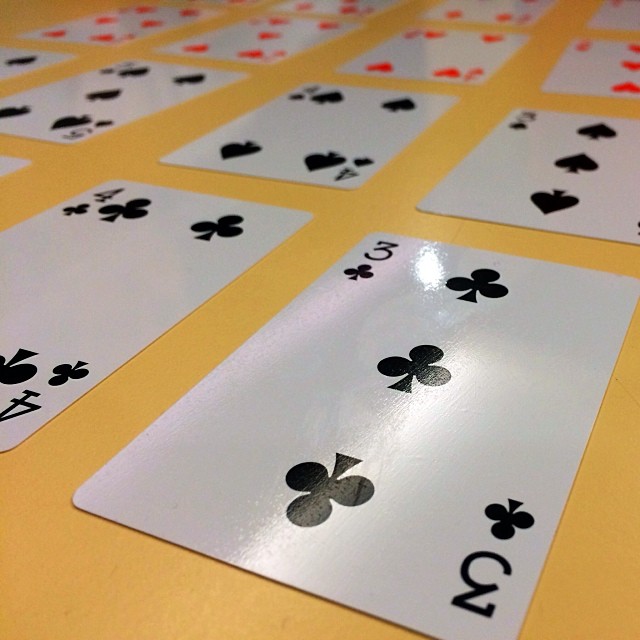The photograph captures a spread of playing cards displayed on a warm, yellow matte table surface. The image is taken from a very low angle, creating a horizon-level view that is slightly tilted downward, allowing a clear view of the cards' faces. The arrangement consists of about 14 to 15 cards, with the 15th being partially cut off in the upper middle left of the frame.

In the foreground, the black cards stand out prominently, organized in two rows. Dominating the center bottom-right of the image is the three of clubs, positioned diagonally from the bottom left to the upper right. To its immediate left lies the four of clubs. Directly above the three of clubs is the three of spades, with the four of spades to its left, followed by the five of spades, and another card that is mostly cut off.

The upper rows feature the red cards, with the row just above the black cards comprising hearts. However, due to the image angle and blur, the numbers on these cards are indiscernible. The topmost row appears to be diamonds, also heavily blurred and partially cut off. The overall composition emphasizes the sharp details of the black cards in the foreground against the softer, more obscured red cards in the background, creating a layered depth effect.